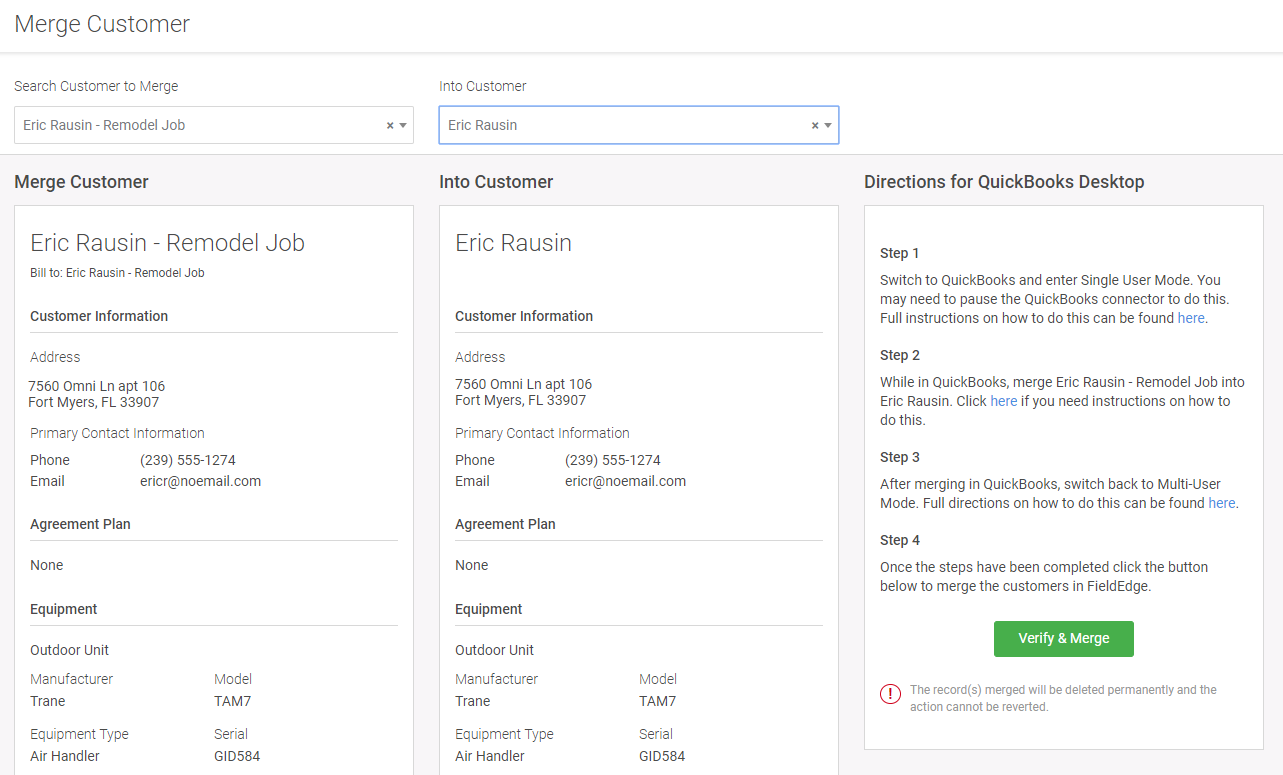At the top left corner in gray text, it reads "Merge Customer," followed by a shadowed gray divider line that spans horizontally across the layout. Beneath this on the left side, there is a small, gray-printed heading that says "Search Customers to Merge," leading into a dropdown menu. The selected option within this menu is labeled "Eric R-A-U-S-I-N – Remodeled Job."

The main interface has a gray background area where, at the top left in bold black font, it reads "Merge Customer." Below this header, a white rectangular section displays more details: at the top, it repeats "Eric R-A-U-S-I-N – Remodeled Job." Underneath, in a very small font, it notes "Bill To: Eric R-A-U-S-I-N – Remodeled Job."

Further down, bold black text introduces the section "Customer Information," separated by a gray line divider. This section includes the address in small black font: "7560 Omni Lane, Apartment 106," followed by "Fort Myers, FL 33907." 

Subsequent information is introduced under the gray title "Primary Contact Information," detailing in black small font "Phone: (239) 555-1274" and "Email: ericr@noemail.com."

Following this, bold black text heads the "Agreement Plan" section, which is blank except for the word "None" underlined by another gray divider line.

The final section titled "Equipment" in bold black font is once again divided by a gray line. It identifies the "Outdoor Unit" with a gray subheading "Manufacturer," beneath which, in small black font, the brand "Trane" is specified.